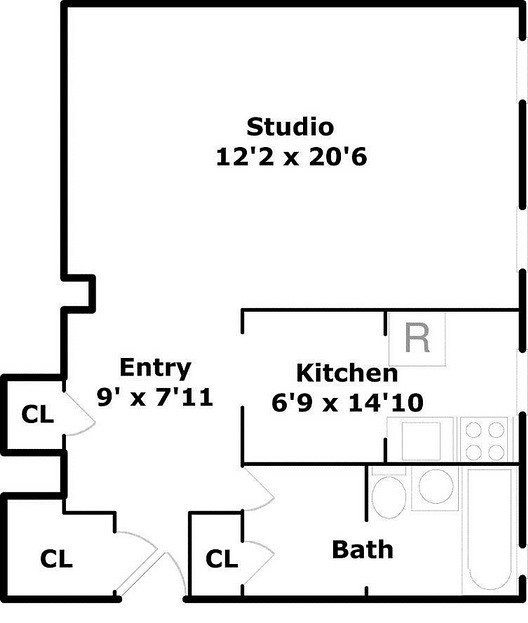This image presents a detailed blueprint of a studio apartment layout, outlined in black. At the top, the blueprint is labeled "Studio 12," with dimensions specified as 12.2 inches by 20.6 inches. Starting from the top left, the entry area is marked, with dimensions of 9 inches by 7.11 inches. Adjacent to the left side of the entry is a small box labeled "CL."

Moving forward from the entry, there is a defined kitchen space measuring 6.6 by 9 inches to 14.10 inches. Below or adjacent to the kitchen area is a designated bath space. The bath area also features a small box on the left, labeled "CL." Additionally, once you exit the bath, there is another "CL" labeled space on the left-hand side. The layout outlines all key elements, highlighting the compact and functional design of the studio apartment.